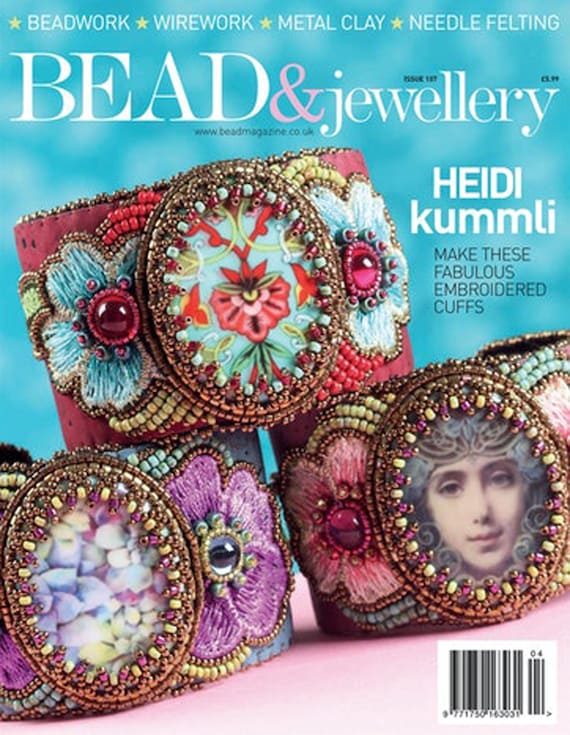This magazine cover features "Bead and Jewelry," highlighted at the top beneath keywords including beadwork, wirework, metal clay, and needle felting. The website listed at the bottom is www.beadmagazine.co.uk. The vibrant cover showcases three elaborate, jeweled cuff bracelets stacked upon each other. 

The top bracelet is adorned with red jewels and incorporates a red and blue floral design with intricate beads and gemstones. The middle bracelet, positioned on the left, has detailed purple embroidery with an array of green, purple, and yellow beads. It features pearl-like stones set within golden circles, embellished with blue flower blossoms and green leaves, transitioning in color from rose to pink, yellow, and various golden hues. 

The bracelet at the bottom right combines red and brown hues and includes red and yellow floral patterns. At its center, it displays a portrait resembling the Mona Lisa. Above the bracelets, the text reads "Heidi Kumli" and underneath, "make these fabulous embroidered cuffs,” emphasizing the craftsmanship of these intricate designs.